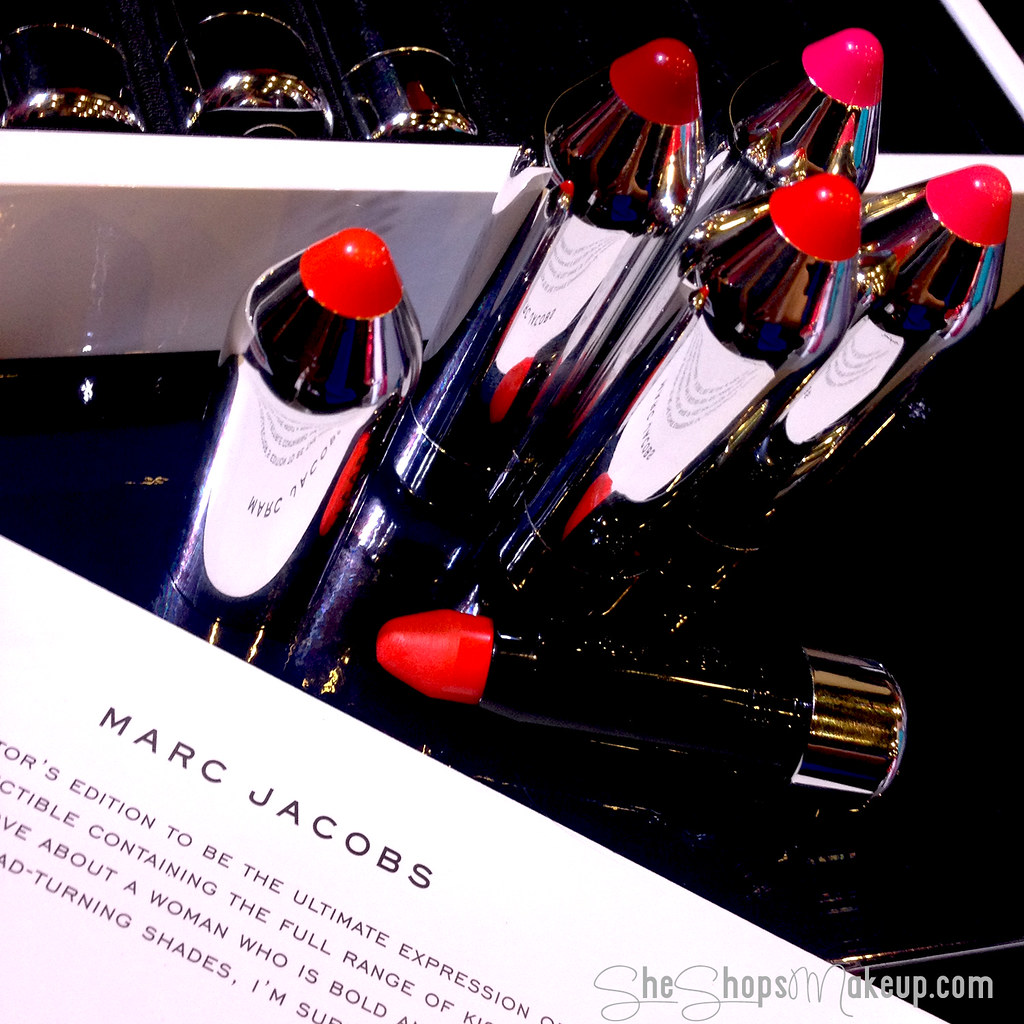This is an ultra-glossy close-up image of cosmetics, featuring five cylindrical lip pencils and a black tube of lipstick, all set against a reflective white wall. The lip pencils are arranged vertically, with colorful tips in shades of red, pink, and dark burgundy, atop shiny silver casings that resemble bullet casings. Each lip pencil stands approximately three to four inches tall and about one inch in diameter. Lying beside them horizontally is a black tube of lipstick, capped with a red top and silver base. Partially visible text printed vertically on the lipstick tube reads "Marc Jacobs", though some lines of text are obscured. In white letters on black, the bottom right corner of the image displays the website SheShopsMakeup.com.